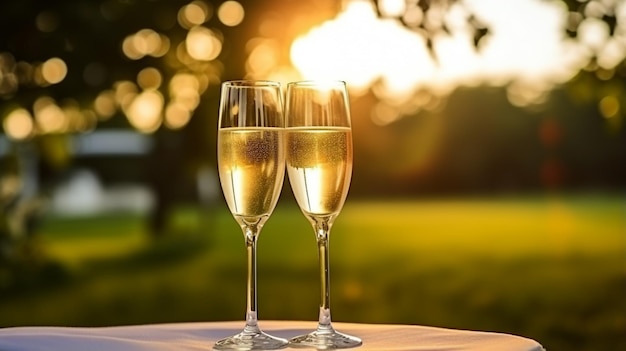In the center of the image, two champagne glasses, filled about four-fifths of the way with bubbling champagne, stand prominently on a table adorned with a white tablecloth. The sunlight, either from dawn or dusk, casts a warm glow through the glasses, creating small light artifacts and reflections. The glasses have a distinct black stripe on their left sides, possibly due to a shadow or object in the background. The backdrop, a blurry natural setting that resembles a park or backyard, features a flat grassland with lush green grass, indicative of a summer day. Several trees populate the background, with two close ones on the left and additional ones where the sun peeks just above. A faint white blur on the left may be a gazebo, adding to the tranquil ambiance. Light filtering through the trees enhances the serene and picturesque scene.